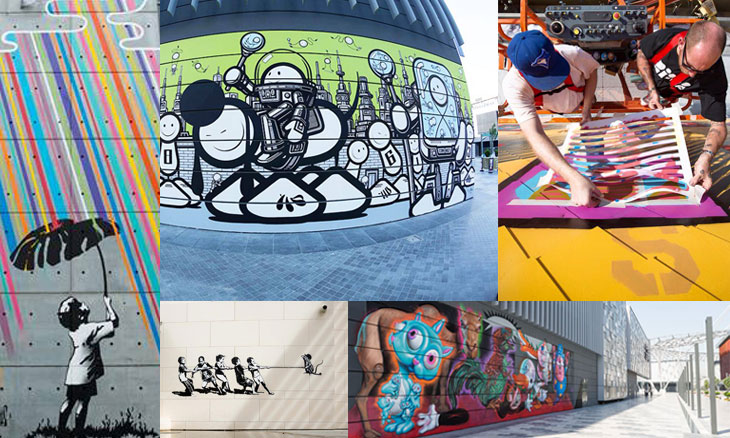The image is a collage of five distinct mural artworks photographed outdoors. The top right picture captures two individuals in safety harnesses on a scissor lift as they apply a stencil to a mural, preparing to paint through perforated paper. Adjacent to this, to the left, is a mural depicting abstract humanoid figures wielding racket-like objects in a fantastical cityscape with a green sky and blue buildings. The leftmost image features a captivating mural of an 8-year-old child standing in grass, holding an enormous leafy umbrella in black and white, shielding against streaks of rainbow-colored rain falling from cloud shapes. Below this, a small mural portrays a playful tug-of-war scene with multiple people pitted against a single rat. Lastly, the bottom right image showcases a vividly colorful mural of cartoon animals along the side of a long sidewalk, including a prominent large blue cat among other cheerful characters.